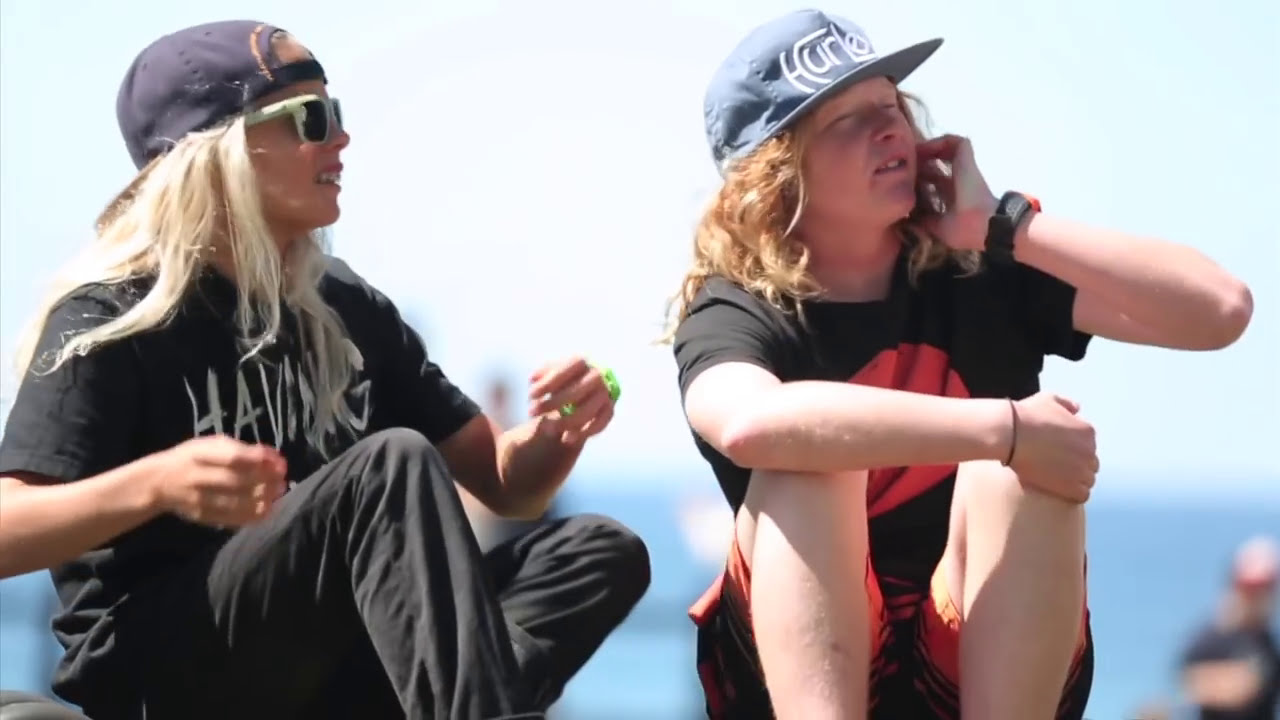The image depicts two young high school-aged individuals, likely sitting on the ground, enjoying a sunny day outdoors. On the left sits a girl with strikingly long, almost white blonde hair. She sports a backwards navy blue baseball cap, light green framed sunglasses with dark black lenses, and a black t-shirt with the word "HAVING" in white capital letters. She is also wearing black pants and has her knees bent up in front of her. Her hands are outstretched in front, and she appears to be speaking or exclaiming something, as her mouth is open.

To her right is a boy with long, curly blonde hair under a light blue "HURLY" cap. His left hand is up to his face as if scratching or perhaps using a phone. He wears a black t-shirt featuring a large red circle design in the center, and red shorts with black stripes. His right arm is draped around his knees, which are bent up similar to the girl's position. His skin appears slightly red, likely from the sun. The background includes a blurred view of other people and a dominant blue hue, suggesting a casual outdoor gathering.